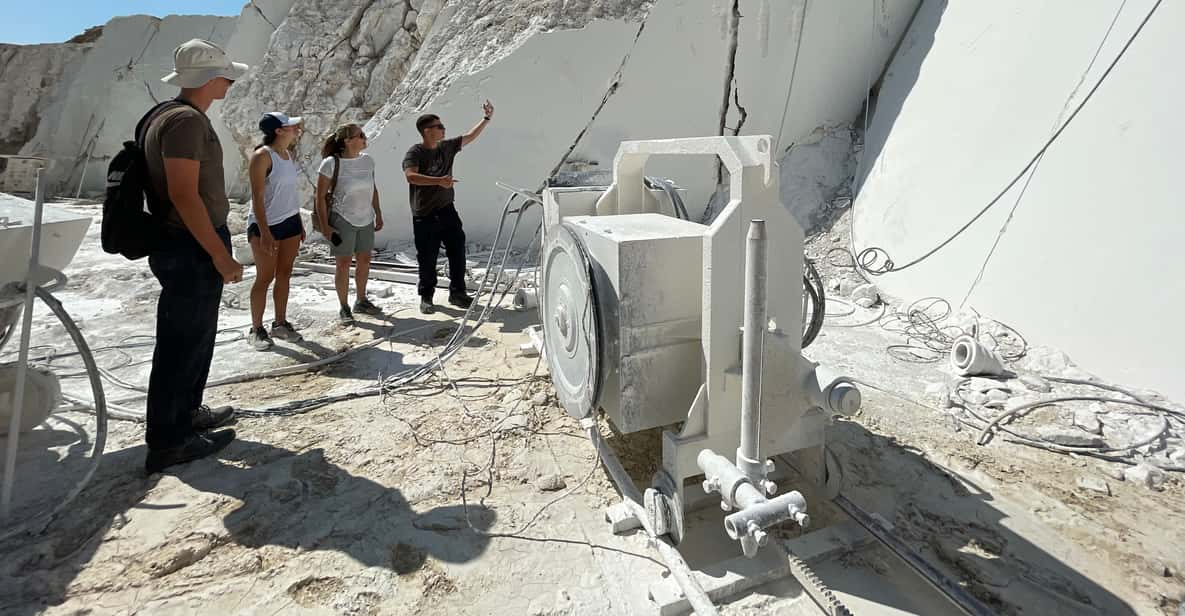The photograph depicts a group of people, likely in their mid-twenties, standing and examining a white marble quarry site under a clear blue sky situated in the top left corner. The person on the far left is a man dressed in a grey shirt and trousers, wearing a grey hat, and carrying a black backpack. To his right are two women; one is dressed in a white shirt and grey shorts, while the other is in a white tank top and grey shorts. On the far right is another man in a black shirt and pants, wearing sunglasses, who appears to be explaining something with his hand raised. The quarry features large, sloping cliff-like structures of white marble. At the center of the image, there is heavy machinery, identifiable by its square or cube-like form with a circular disk and multiple cables connected to it, possibly used for extracting marble.